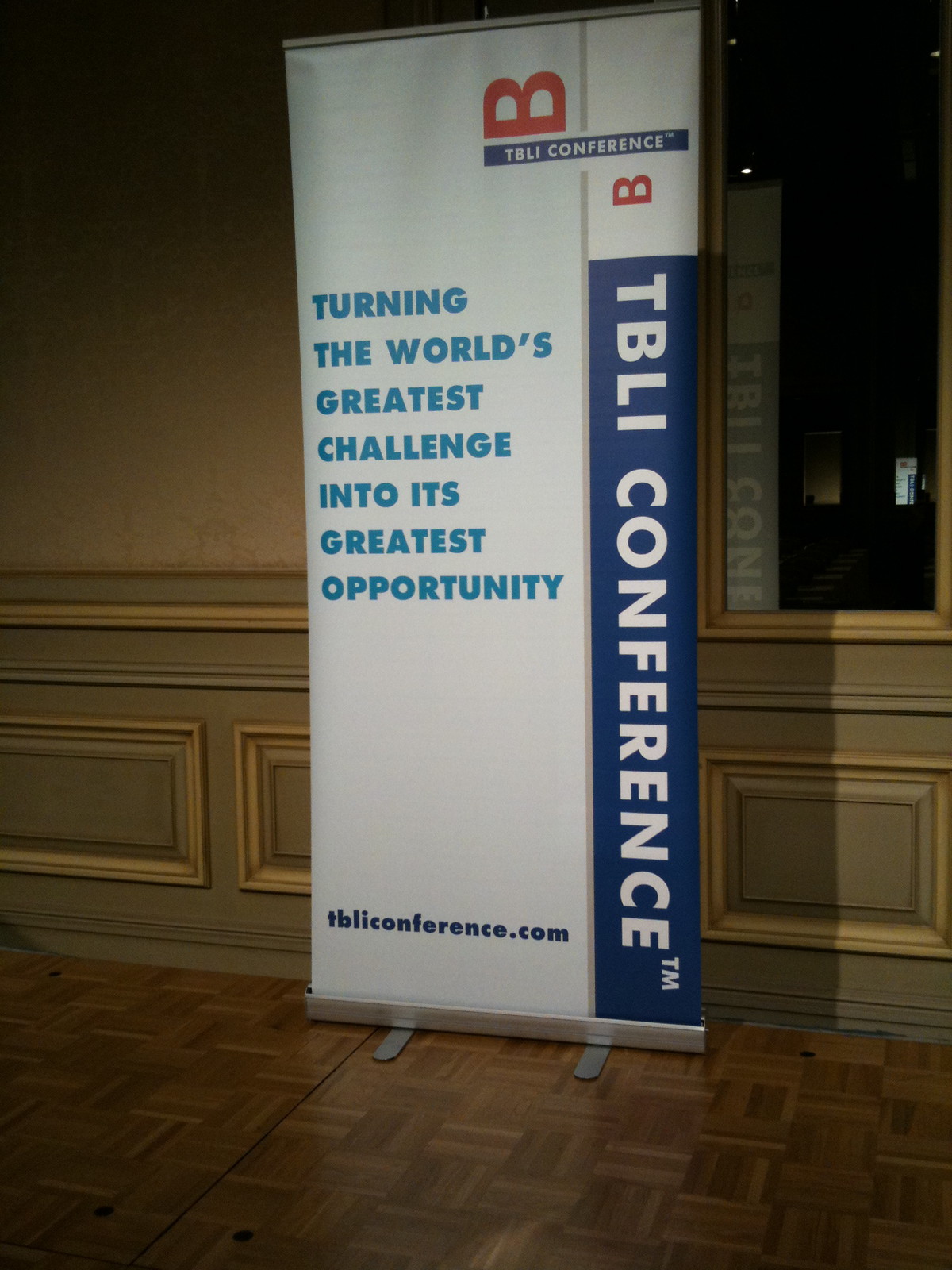The image captures a tall, vertical rectangular sign prominently displayed in a drab indoor room with light brownish walls and a less appealing olive green trim. The room has parquet flooring, and the sign is mounted on two silver metal legs. Positioned on the right, the sign says "TBLI Conference" in white font on a vertical blue bar. To the left, against a white background with a very light blue tint, the sign reads, "Turning the World's Greatest Challenge into Its Greatest Opportunity" in blue text. At the bottom of the sign, the website "TBLIConference.com" is displayed in dark text. Additionally, there are two large, sideways red "B" letters situated near the top and bottom right corners of the sign, with another blue horizontal bar inscribed with "TBLIConference" in white text below the upper "B." The background wall bears fancy molding at the base, and to the right of the sign, there is a large vertical rectangular window or possibly a mirror with a dark reflection, suggesting it could be nighttime outside.